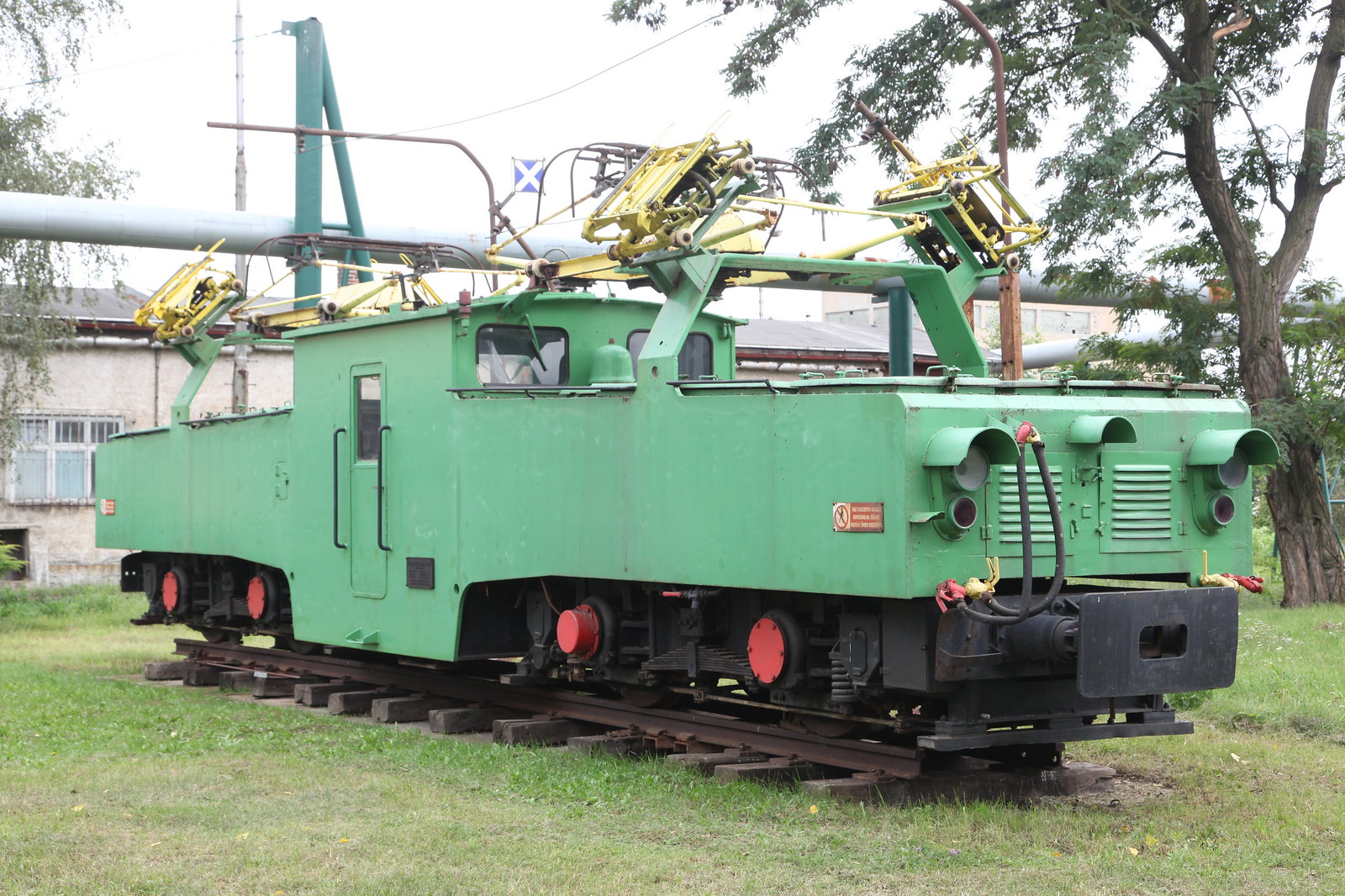A peculiar green machine is prominently displayed outdoors on a small section of railroad track, surrounded by grass and trees in the background. The machine, reminiscent of a tank without a cannon due to its boxy structure, appears to be a specialized piece of equipment designed for maintaining railroad tracks. Its purpose is likely to clear debris from the tracks to ensure safe passage for trains. The display setting, featuring a cross-sectional piece of track rather than a full railroad, suggests an educational or demonstrative intent, showcasing the machine’s role in railway maintenance.